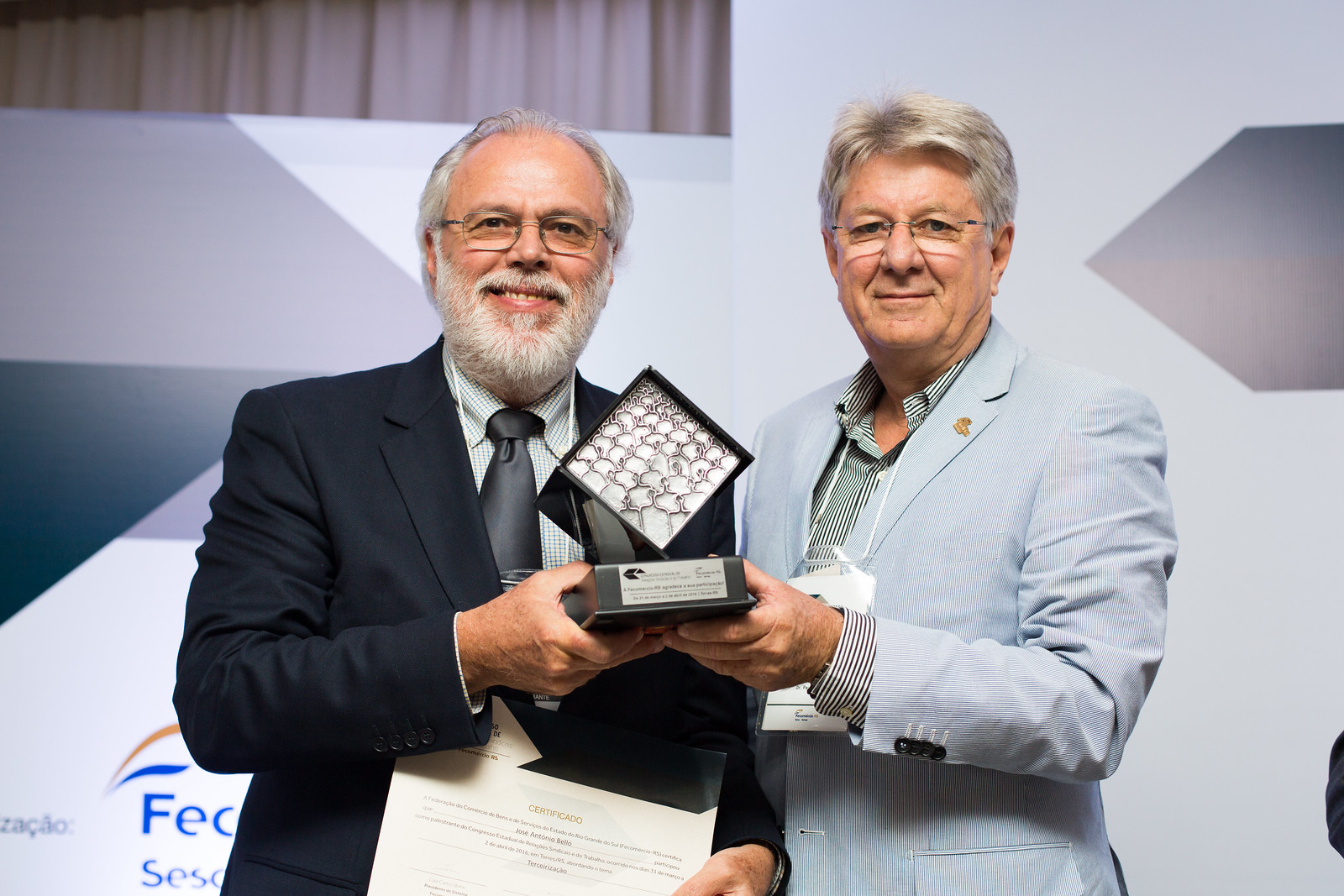This vibrant color photograph captures a celebratory moment at an event with two elderly Caucasian gentlemen standing shoulder-to-shoulder, facing the camera and smiling. Each, with one hand, is holding an award between them, which is diamond-shaped and mounted on a plinth with a gold plaque. The man on the left, who has grayish-white hair along with a beard and mustache, is dressed in a black suit with a white shirt and a black tie. He is additionally holding a certificate in his left hand. He sports wireless rimmed glasses. The man on the right, who has similar grayish-white hair but is clean-shaven, is dressed in a blue and white striped jacket over a darker blue pinstripe shirt. He also wears glasses and has a lanyard with a name tag around his neck. Both men exude a sense of accomplishment, underscored by their smiles and the prestigious award they hold. The image further includes stage elements such as backdrops and curtains, indicating that this significant moment is part of a formal event.